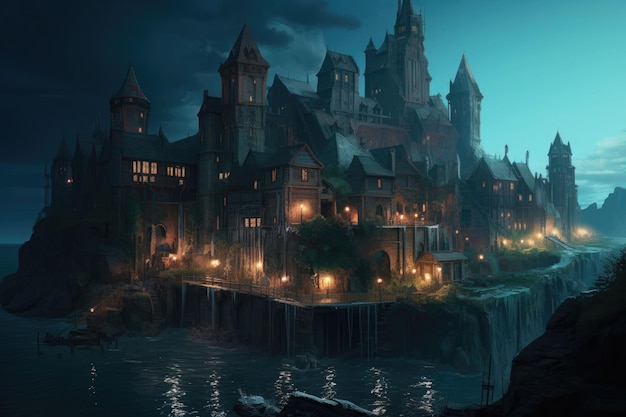The image depicts a highly detailed, digitally rendered, large castle structure that combines elements of both a cathedral and a traditional castle, evoking a gothic aesthetic. It features six tall towers with a mix of architectural styles—some resembling castle turrets while others look like church steeples, all culminating in pointed roofs. The building is illuminated with glowing orange lights from windows and numerous street lamps surrounding the area, casting a warm glow on the stonework. Situated on an island or peninsula, the structure is edged by calm waters on the left side, reflecting the serene environment. A pathway lined with lighted lamps winds around the island. The night sky above features a mix of blue and dark clouds, creating a dramatic atmosphere. Trees and a cliff can be observed in the scene, framing the majestic view of this grand, castle-like edifice.